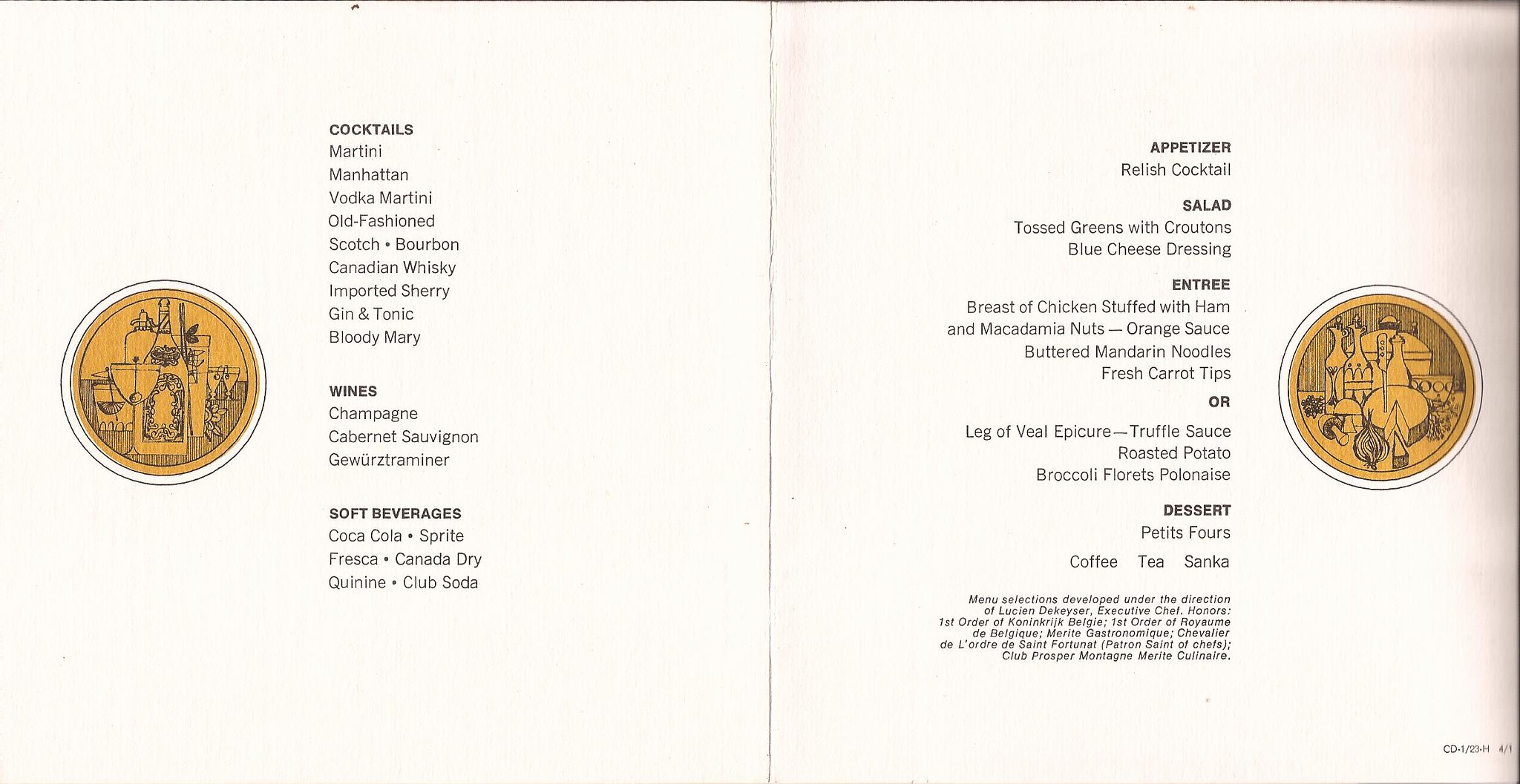The image portrays a specialty menu meticulously presented as an open book, with a seam dividing its two pages. Each page is adorned with a rustic, wooden-colored seal or emblem positioned in a circle at the outer margins. The left seal features a prominent wine bottle, complemented by scattered images of wine glasses and martini glasses, all hand-drawn or sketched with a delicate touch. The seal on the right showcases a variety of wine bottles with different stoppers, also illustrated in a detailed, hand-drawn style.

The left page of the menu lists a selection of cocktails in a small, refined font, including Martini, Manhattan, Vodka Martini, Old Fashioned, Scotch and Bourbon, Canadian Whiskey, Imported Cherry, Gin and Tonic, and Bloody Mary. Below the cocktails, an array of wines and champagne is presented, with options such as Cabernet Sauvignon and Gewurztraminer. The beverage section continues with a variety of soft drinks like Coca-Cola, Sprite, Fresca, Canada Dry, Quinine Club, and Soda, organized into three rows and two columns.

On the right page, the menu offers a tempting array of appetizers, salads, entrees, and desserts. The appetizer section lists a Relish Cocktail Salad featuring tossed greens, croutons, and blue cheese dressing. For the entree, options include a Breast of Chicken stuffed with Ham and Macadamia Nuts drizzled with Orange Sauce, accompanied by Buttered Mandarin Noodles and Fresh Carrot Tips, or a Lake of Fuel Epicure served with Truffle Sauce, Roasted Potatoes, and Broccoli Florets. The dessert options feature 54's along with Coffee, Tea, and Cinca. The bottom right corner of this page contains some indiscernible writing, possibly in French, adding an additional touch of elegance to the menu.